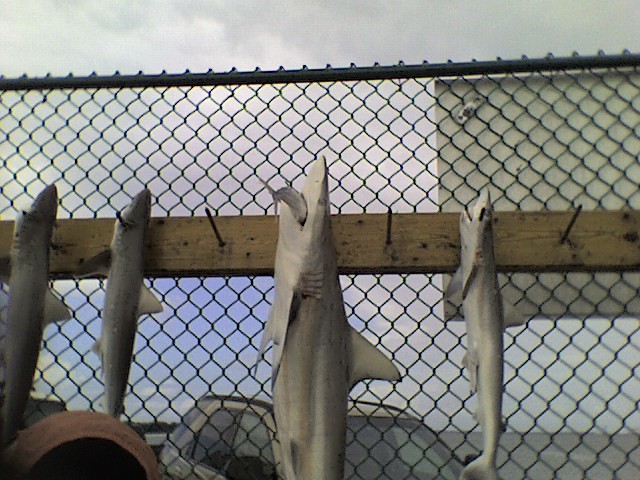The photograph captures a grim display of several shark carcasses nailed to a wooden plank, which is itself fastened to a black chain-link fence with a solid top bar. The sharks, numbering five in total, are positioned with their mouths fully open and facing upwards, impaled through their gills by nails jutting outward from the board. The central shark is the largest, flanked on each side by two smaller sharks roughly the length of a person’s forearm. To the far left of the image is an additional small shark, while an empty nail awaits on the far right. The whole scene is captured under dim, dingy lighting, complete with some film grain effect. The backdrop features a cloudy, overcast sky with just a small patch of blue. A beige SUV is partially visible at the bottom of the image, behind the fence. On the top right, a white plastic sign is affixed to the other side of the fence, though its text remains hidden from view. No people or additional structures are present in the photograph.